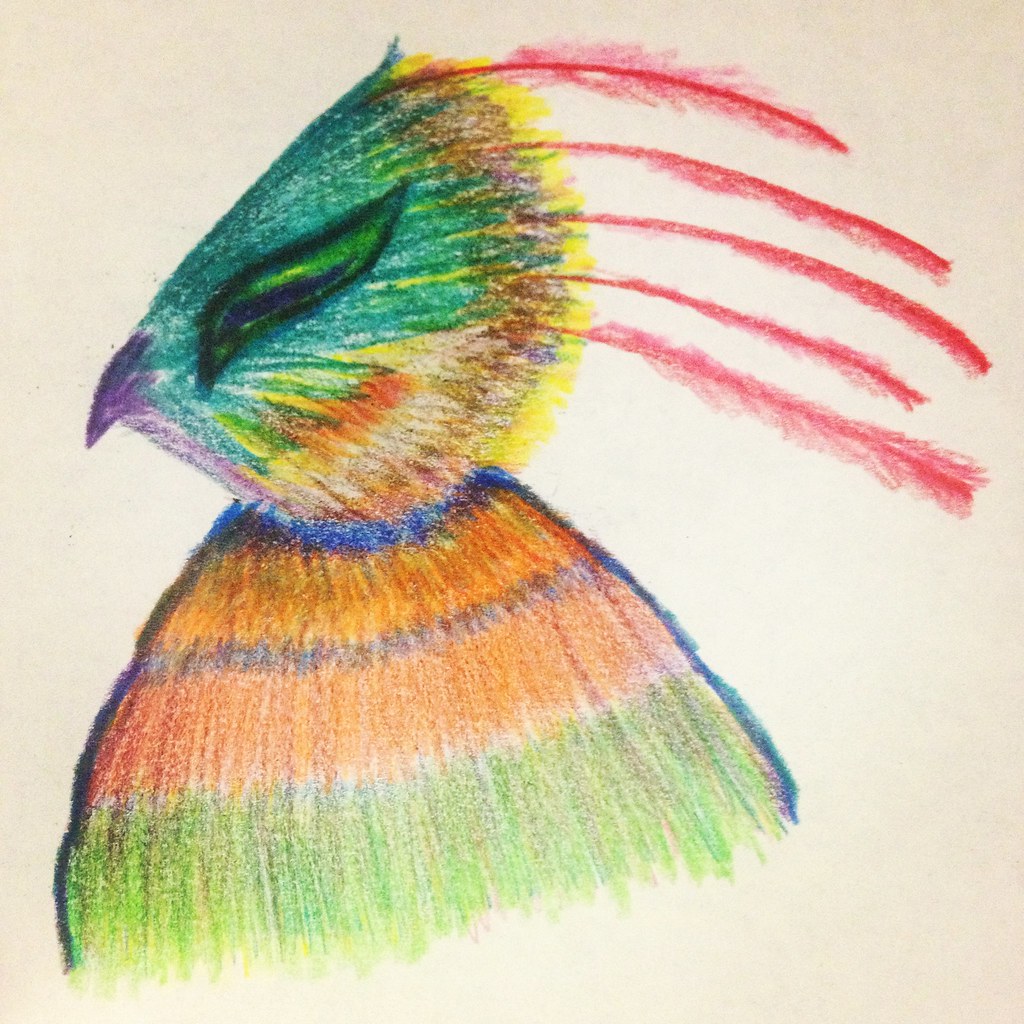This vibrant drawing depicts a bird created meticulously with colored pencils, showcasing a rich, layered texture. The artist skillfully blended a multitude of hues, including greens, yellows, oranges, reds, purples, and blues. These colors harmoniously transition and meld into one another, creating an intricate and dynamic visual effect. The detailed application of each layer highlights the bird's feathers and form, adding depth and dimension to the artwork. The vivid palette and thoughtful blending techniques make this a captivating and unique portrayal of avian beauty.